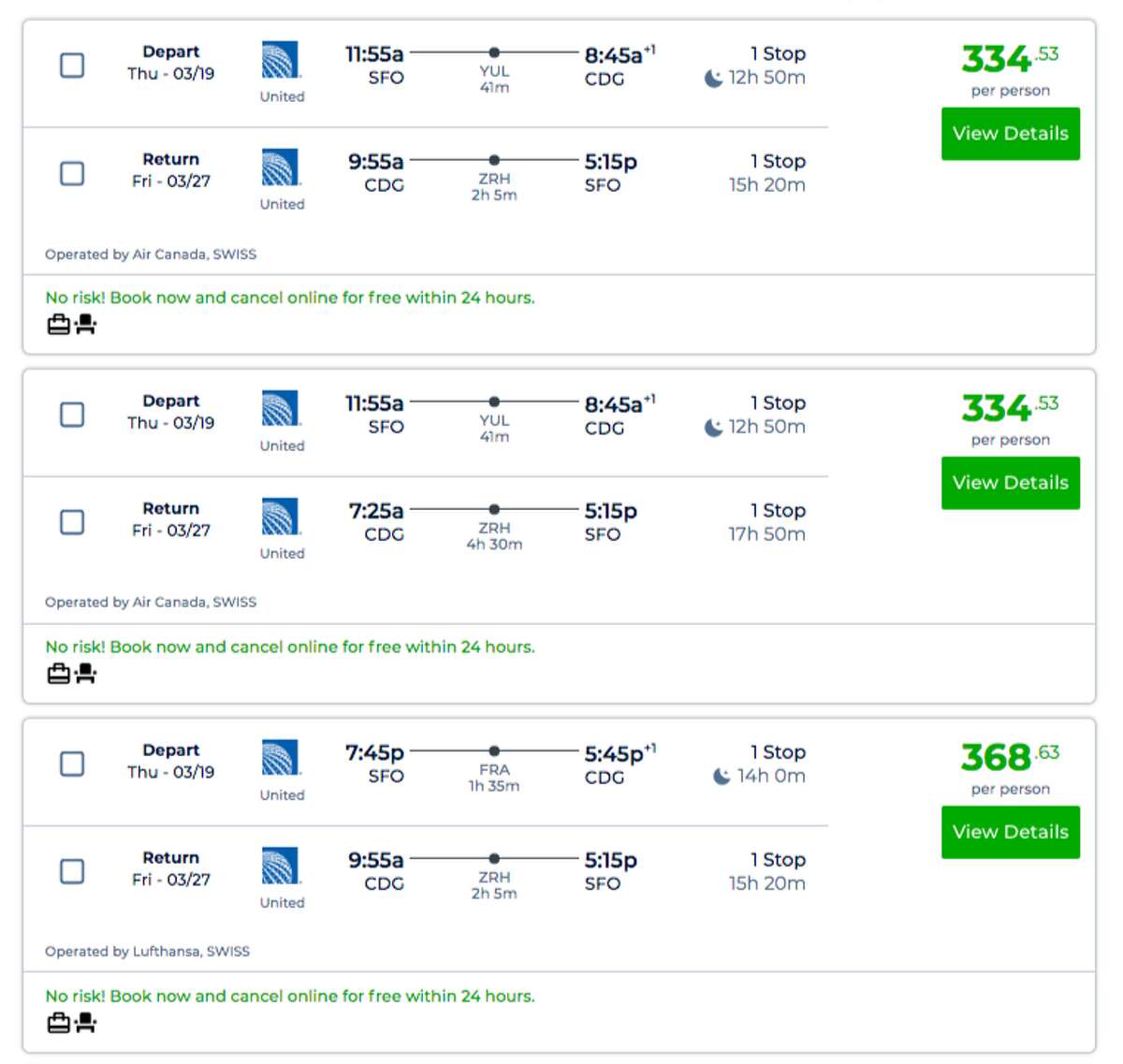This image is a screenshot from a travel website displaying flight options for a trip. There are three different fare options for round-trip flights, all with the same departure and destination airports.

1. **First Option:**
   - **Departure:** Thursday, March 19th at 11:55 AM from San Francisco International Airport (SFO) on United Airlines.
   - **Arrival:** 8:45 AM the following day at Charles de Gaulle Airport (CDG) in Paris with one stop.
   - **Return:** 9:55 AM from CDG on United Airlines, landing at 5:15 PM in SFO with one stop.
   - **Price:** $334.53 per person.
   - **Features:** Includes a green "View details" button. The booking is risk-free with free cancellation within 24 hours.

2. **Second Option:**
   - Identical flight details to the first option (same departure, arrival times, and airlines), but with longer layovers.
   - **Price:** $334.53 per person.
   - **Features:** Includes a green "View details" button. The booking is risk-free with free cancellation within 24 hours.

3. **Third Option:**
   - Identical flights (same departure, arrival times, and airlines) but with different layovers compared to the other options.
   - **Price:** $368.63 per person.
   - **Features:** Includes a green "View details" button. The booking is risk-free with free cancellation within 24 hours.